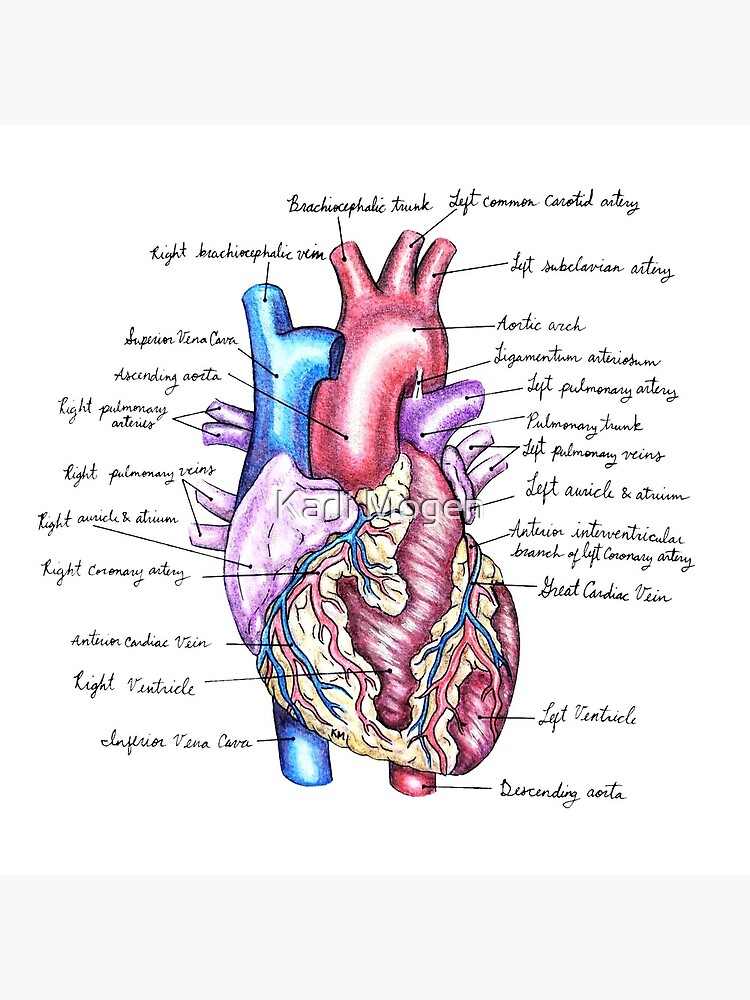This is a detailed drawing of an anatomically correct human heart on white printer paper, rendered in colored pencil. The heart is intricately illustrated with veins and arteries in blue and red, while some regions showcase a mix of colors, including a purple section below the primary vessels. The drawing meticulously highlights parts of the heart with numerous arrows pointing to various sections, each labeled in black cursive handwriting. The labeled components include major arteries like the brachiocephalic trunk, left common carotid artery, and left subclavian artery, as well as veins such as the right brachiocephalic vein. Structural details are also annotated, including the aortic arch, pulmonary trunk, left pulmonary veins, left auricle and atrium, anterior interventricular branch of the left coronary artery, great cardiac vein, left and right ventricles, descending aorta, and inferior vena cava. The heart is surrounded by tissues, possibly representing muscle or fat, adding to the complexity and realism of the diagram.